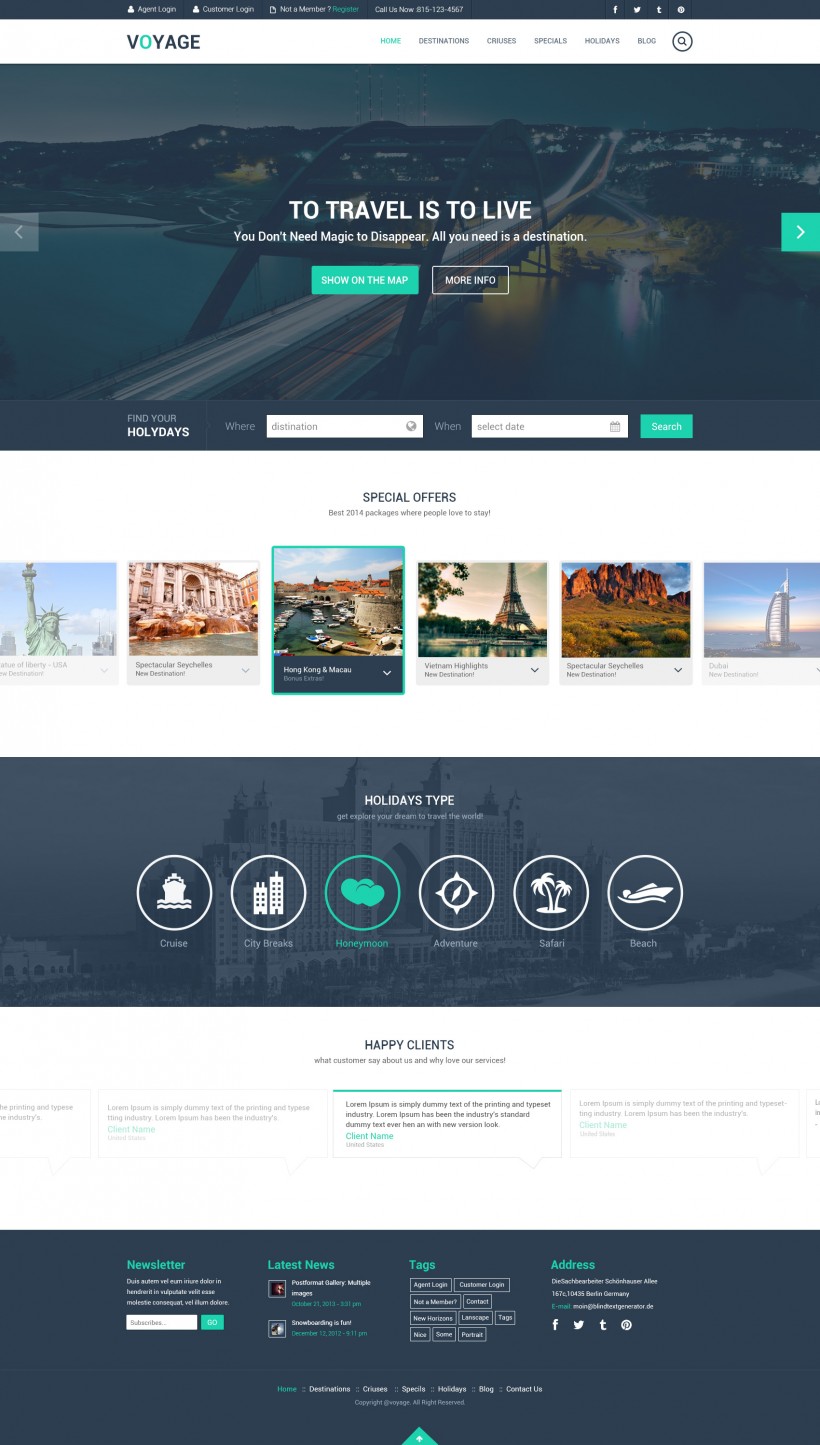This image appears to be a stitched-together screenshot of a webpage, possibly taken on a desktop or tablet. The screenshot encompasses the entire webpage, from the top banner down to the footer, capturing all details including navigation buttons and the copyright notice, although the year of the copyright is not indicated, making it difficult to ascertain when the page was published or last updated.

The webpage belongs to a company called "Voyage," evident from its simple sans-serif logo wherein the 'O' is highlighted in a lighter teal color. The page emphasizes travel packages and also offers cruises, though "cruises" is misspelled as "CRIUSES," suggesting that this might be a draft or a template that has yet to be finalized.

A prominent header across the top of the page features the travel-inspired quote, "To travel is to live. You don't need magic. Disappear. All you need is a destination." Below this motivational line are two buttons labeled "Show on the map" and "More info," which add a rather cheesy touch to the otherwise serious travel theme.

The central section of the page is interactive, allowing users to select a destination and desired travel dates, and then search for corresponding packages. However, there is a typo in the phrase "find your holy days," where "holidays" is incorrectly spelled with a 'Y.'

Further down, the page advertises various special offers, best travel packages from 2014, and popular accommodation options, presented in a tabbed format which users can navigate through. These elements collectively indicate the website's purpose of attracting potential travelers through various enticing offers and inspirational quotes.